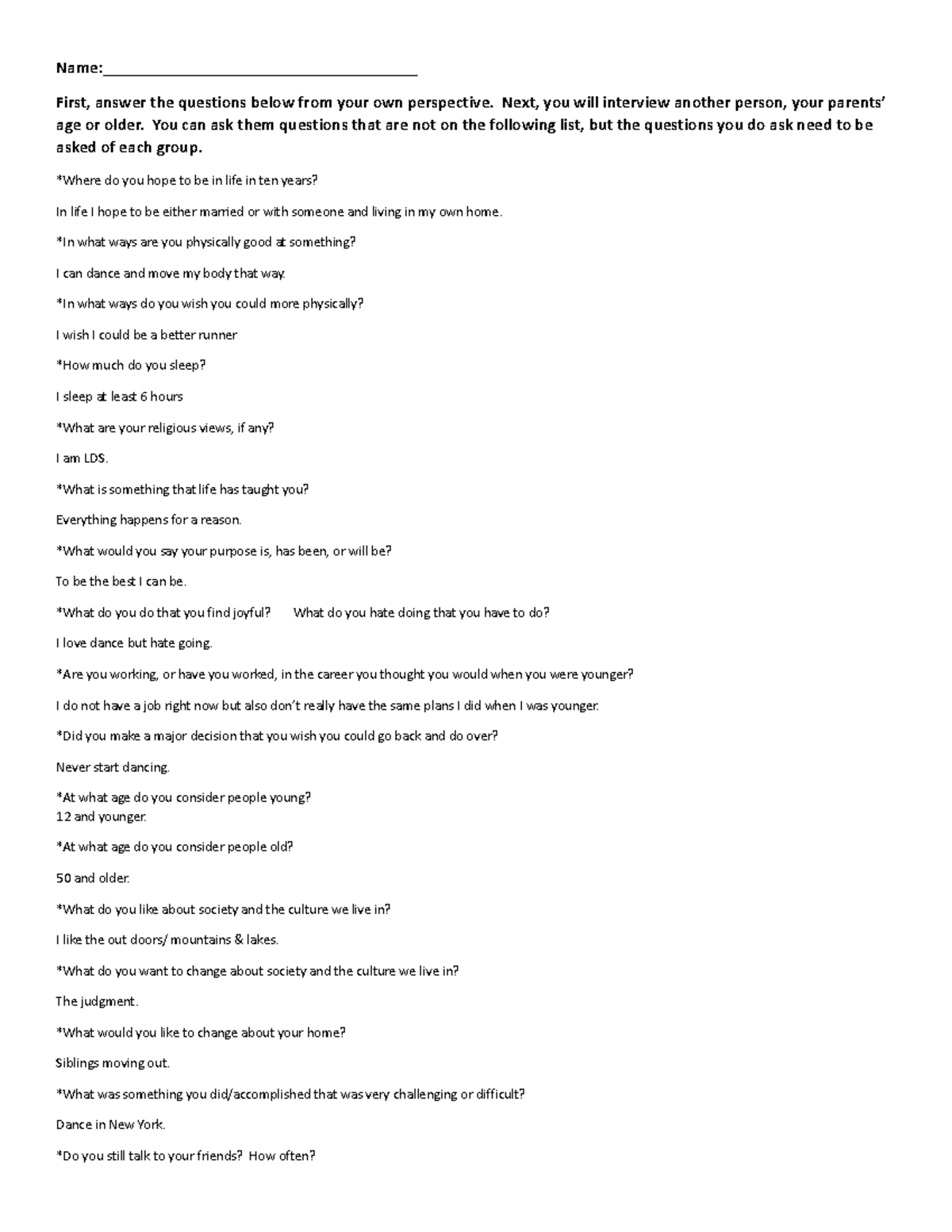The image features a large block of text, left-justified against a white background with black font. At the top of the text, there's a heading labeled "Name: ___," followed by a black line where one can fill in their name. Below the heading, the text outlines a set of personal reflection questions for an exercise.

The instructions state: "First, answer the questions below from your own perspective. Next year, we will interview another person your parents' age or older. You can ask them questions that are not on the following list, but the questions you do ask need to be asked of each group." Below this, a series of question and answer segments are listed:

1. **Where do you hope to be in life in ten years?**
   - *In ten years, I hope to be either married or with someone and living in my own home.*

2. **In what ways are you physically good at something?**
   - *I can dance and move my body in that way.*

3. **In what ways do you wish you could move more physically?**
   - *I wish I could be a better runner.*

4. **How much do you sleep?**
   - *I sleep at least six hours.*

5. **What are your religious views, if any?**
   - *I am LDS (Latter-day Saint).*

6. **What is something that life has taught you?**
   - *Everything happens for a reason.*

7. **What would you say your purpose is, has been, or will be?**
   - *To be the best I can be.*

8. **What do you do that you find joyful? What do you hate doing that you have to do?**
   - *I love dancing but hate going to work.*

9. **Are you working or have you worked? Is your career what you thought you would have when you were younger?**
   - *I do not have a job right now, and my career plans have changed from what I thought they would be when I was younger.*